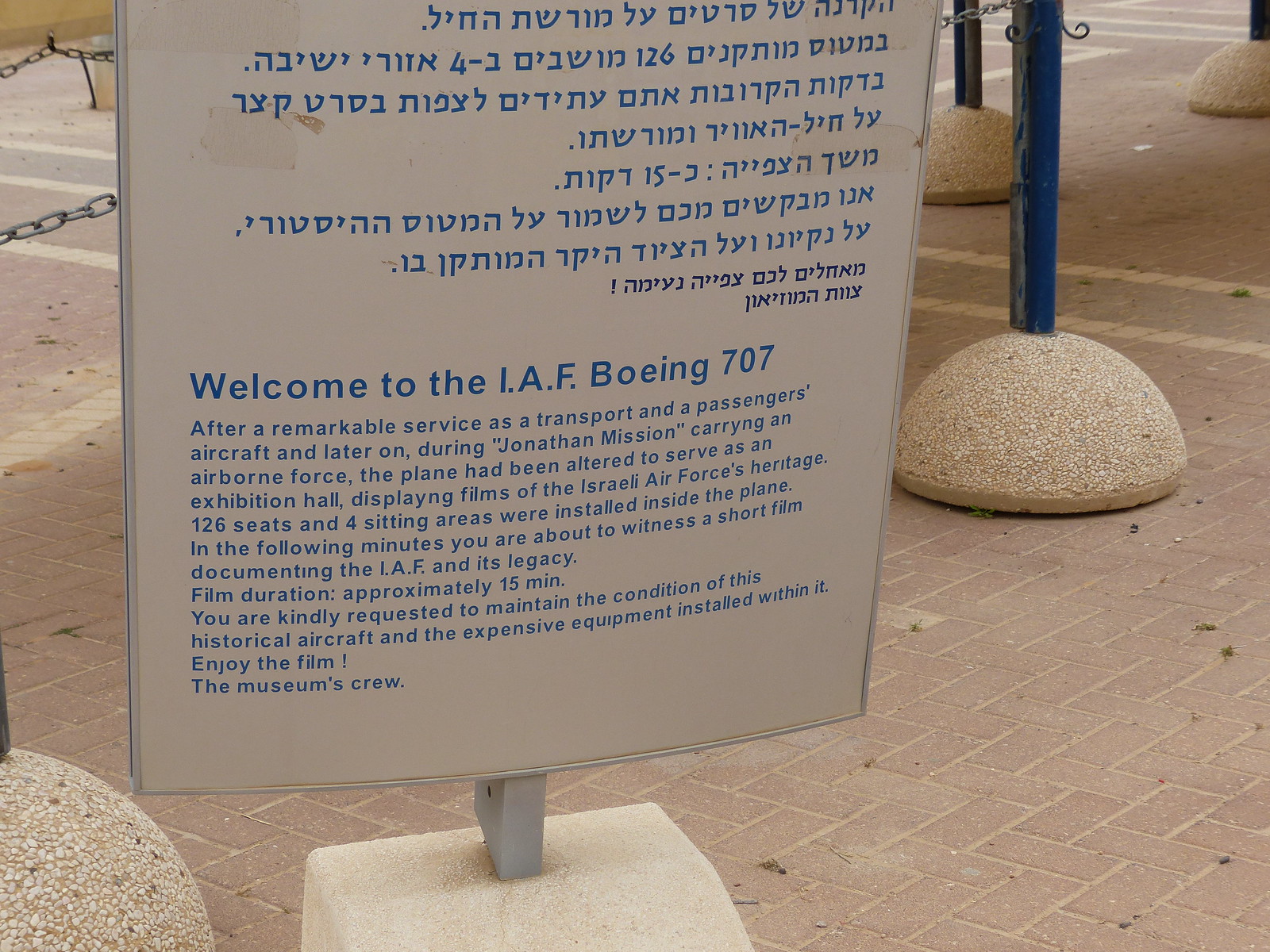The image captures an outdoor scene, likely in a town center or museum setting, with a focal point being a detailed white rectangular sign mounted on a sturdy stone base. The sign, bordered with metal, displays information in both an undecipherable language, possibly Hebrew, and English, with the latter prominently stating, "Welcome to IAF Boeing 707." The English text elaborates on the aircraft’s history, mentioning that after serving as a transport and passenger aircraft, and later in Jonathan's mission carrying airborne forces, the Boeing 707 was converted into an exhibition hall. This hall features 126 seats and four sitting areas where visitors can view films detailing the heritage of the Israeli Air Force. The descriptive text ends with a polite request to maintain the historic aircraft and its equipment, adding a note of gratitude from the museum crew. The surroundings include a brick or brown stone walkway adorned with metal posts and chains, adding to the exhibit-like atmosphere of the scene.